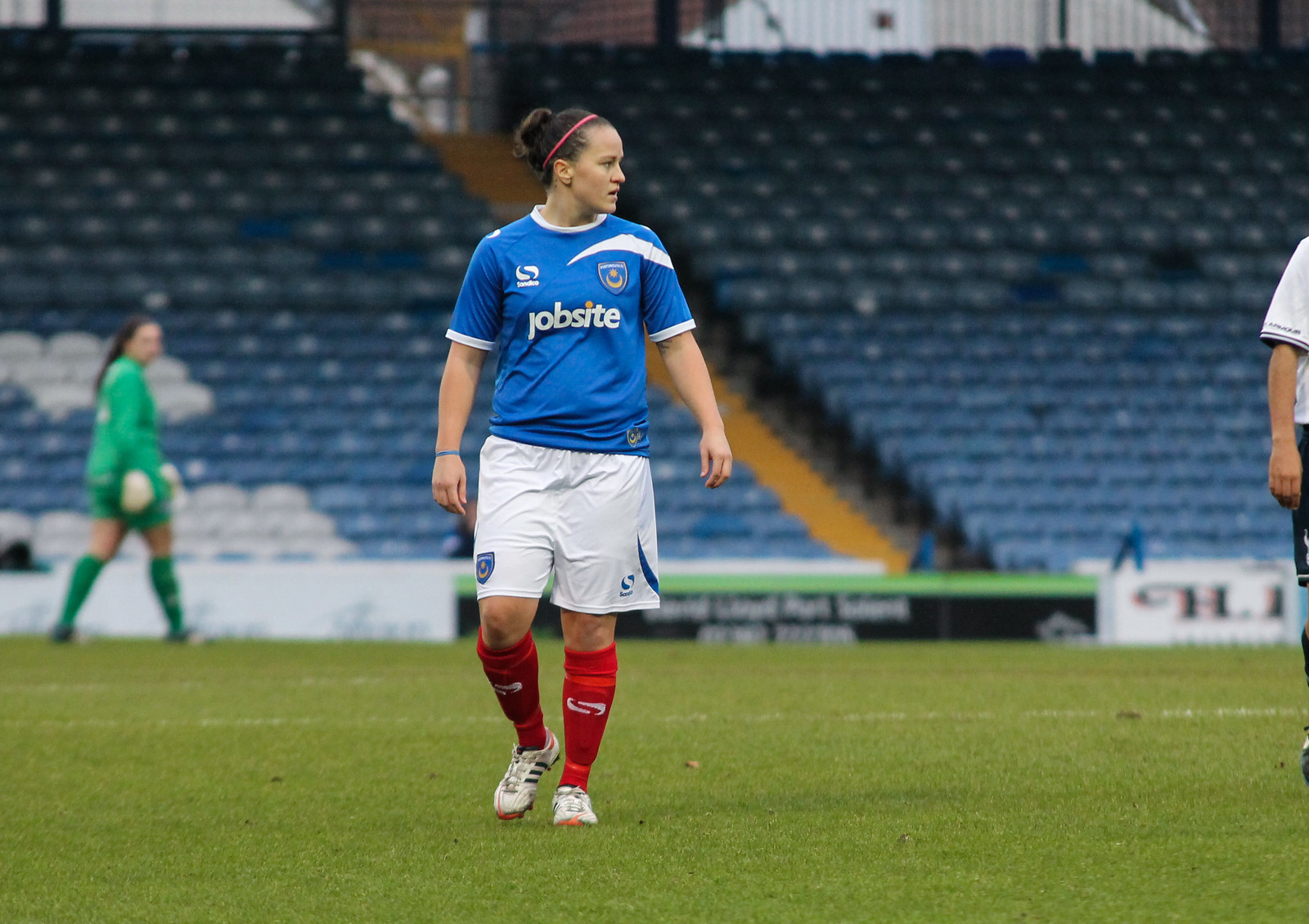In the image, a female footballer, the primary focus of the photograph, is depicted during what appears to be a pregame or practice session, as the stands behind her are entirely empty. She is wearing a blue jersey with the word "Jobsite" in white letters, white soccer shorts, red shin guards, and white cleats that seem to be Adidas. This player is standing on a well-maintained turf field, marked with faint white lines. To her left (our right), there's an arm of someone, possibly a referee, dressed in a white shirt and black shorts, just peeking into the frame. To her right (our left), in the background, is an assumed goalie, clad in an all-green outfit—green long sleeves, shorts, shin guards, and white gloves—though the goalie appears blurry. The empty stands in the background are predominantly blue, with sections of white seats and a distinctive orange aisle cutting through them at a 45-degree angle. Below the stands, blurry advertisements can be seen.